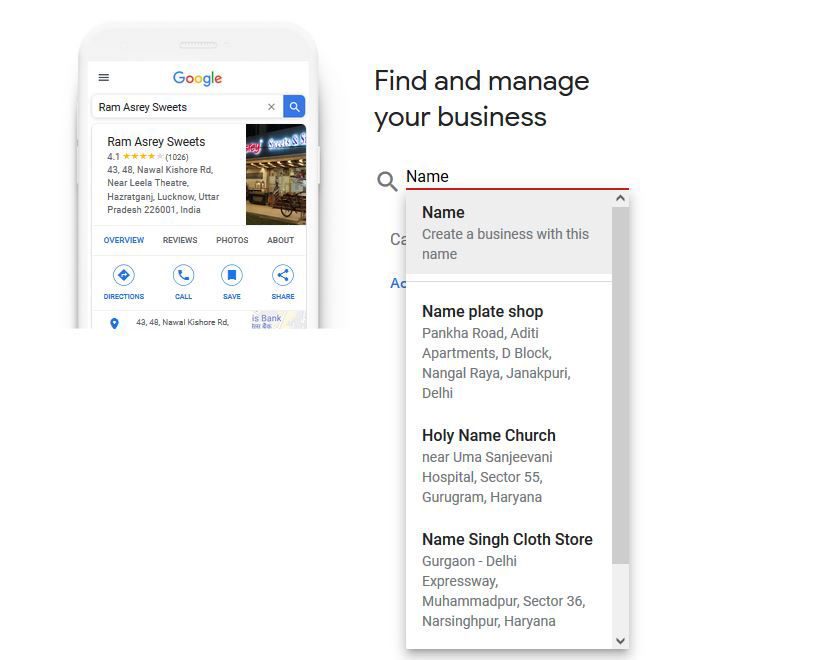The image displays a partial view of a mobile phone screen featuring a Google Maps search result for "Ram Azry Suites" in India. The hotel is located in Hazratganj, Lucknow, Uttar Pradesh, with the postal code 226001. The listing indicates that Ram Azry Suites has garnered a 4.1-star rating based on approximately 1,000 reviews. The visible portion of the phone screen highlights several interactive options: 'Overview' (which is currently selected), 'Reviews', 'Photos', and 'About'. Additionally, buttons are present for obtaining directions, making a call, saving the location, or sharing the page. On the right side of the image, separate from the phone screen, a text prompt about managing a business listing is visible, with contextual examples like "nameplate shop," "holy name," and "sing cloth store." The image's layout and text suggest functionality akin to a business management or directory service interface.